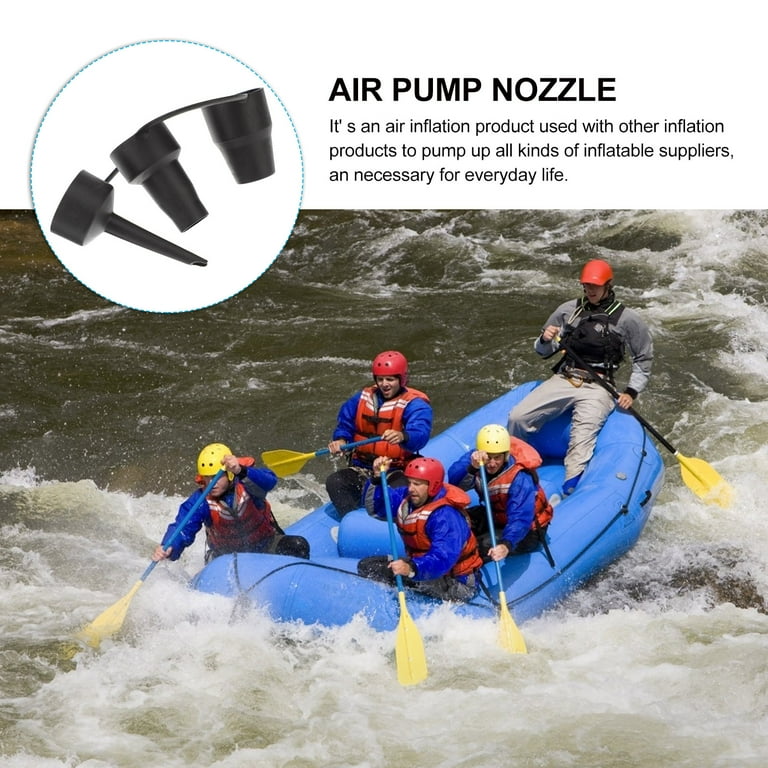This photograph is part of an advertisement for an air pump nozzle. At the top of the image, "Air Pump Nozzle" is prominently displayed in bold black font. Beneath this, three lines of black text explain that it is an air inflation product used with other inflation products to pump up all kinds of inflatable supplies, asserting its necessity for everyday life. To the left side, there's a blue dotted circle featuring the air pump nozzle with three interconnected parts at the top.

The lower portion of the image captures an intense white-water rafting scene. A large, blue inflatable raft navigates the choppy, foamy water. Onboard, five people are outfitted in orange safety vests and either red or yellow helmets, with the majority also wearing long-sleeved blue jackets. The people in the foreground are holding paddles with blue handles and yellow blades. In contrast, the man positioned at the back of the raft sports a gray jacket, khaki pants, and a red hat, and uses a paddle with a black handle and yellow blade. The scene vividly highlights the rough, fast-moving waters around the raft, emphasizing the thrill of the adventure.